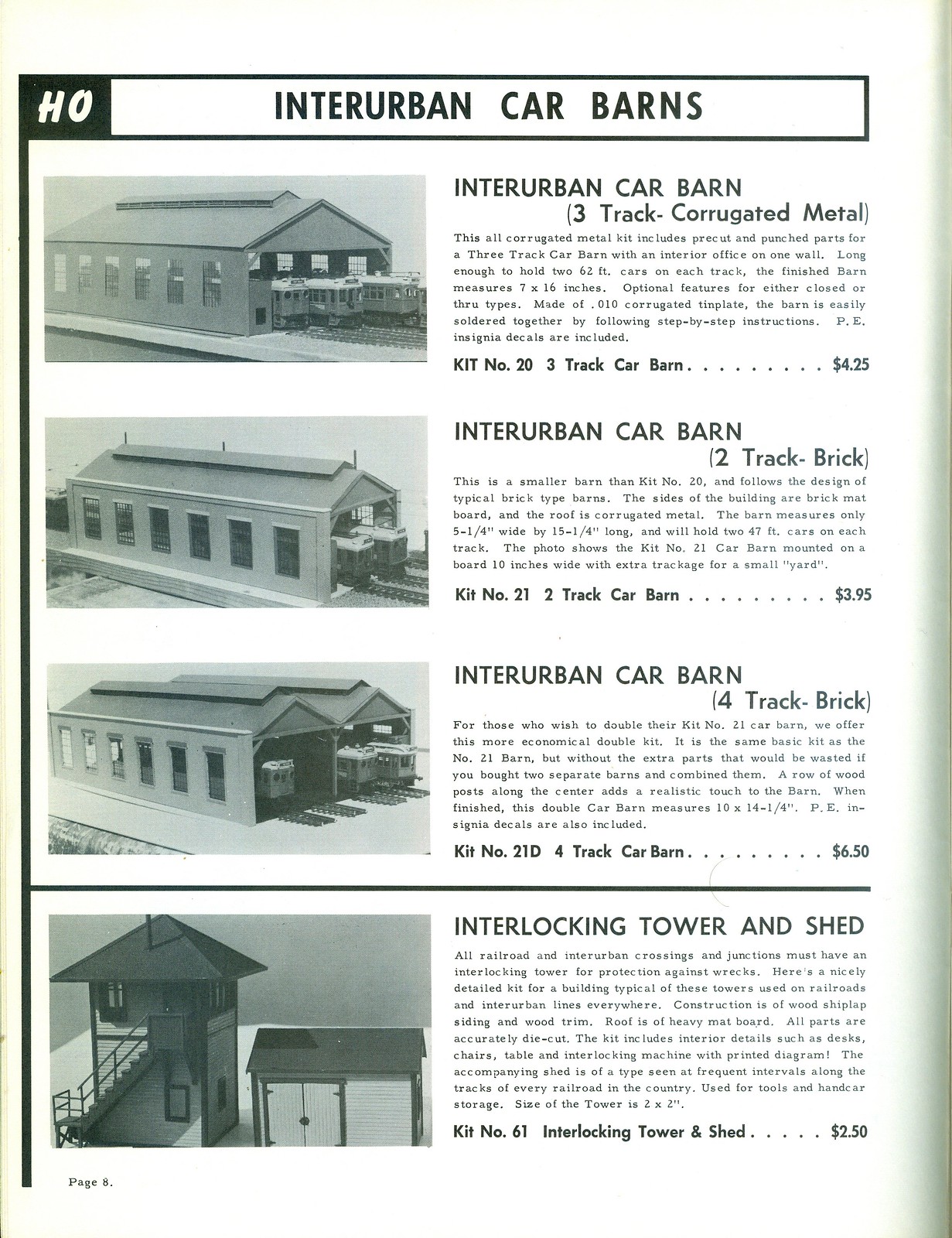This black-and-white image appears to be a vintage magazine advertisement or catalog page, likely from the 1940s or 1950s, showcasing model railroad buildings. The top left corner features a black square with the letters "HO," denoting the scale of the model pieces. The main heading reads "Interurban Car Barns," highlighting various miniature buildings designed to house model trolley cars. Four items are detailed with prices: 
1. **Interurban Car Barn (3-track corrugated metal)** - $4.25
2. **Interurban Car Barn (2-track brick)** - $3.95
3. **Interurban Car Barn (4-track brick)** - $6.50
4. **Interlocking Tower and Shed** - $2.50

The three car barns are illustrated with photographs depicting long structures suitable for different track configurations. The interlocking tower and shed resemble a small guard tower adjacent to a shed. The page is numbered 16, suggesting it's part of a larger HO scale model product catalog. The advertisement, with its grayscale tones and distinct sections, gives a nostalgic glimpse into the model railroading hobby of the mid-20th century.